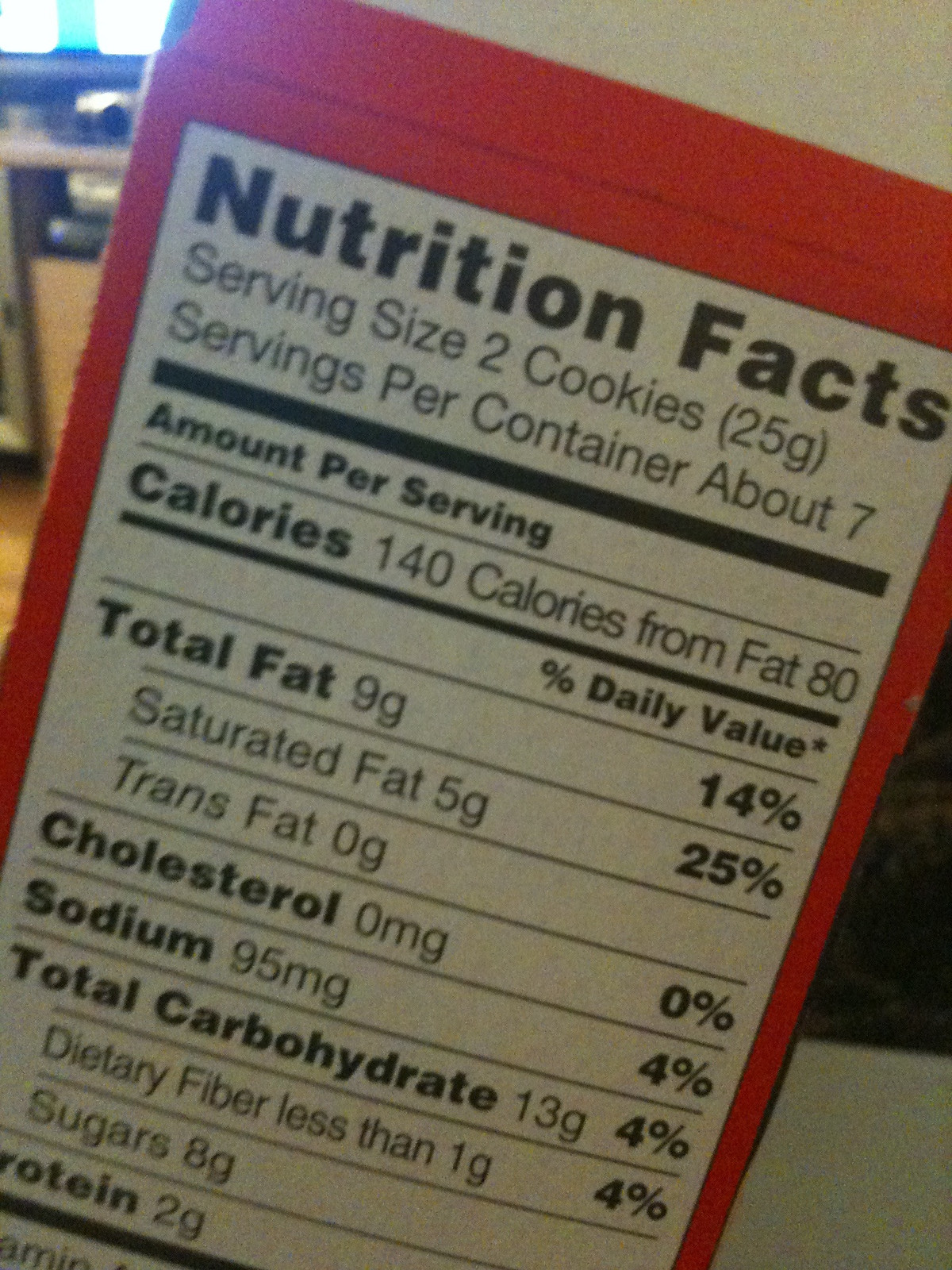This detailed close-up photograph showcases a Nutrition Facts label on a red cardboard box, which is tilted at approximately a 20-degree angle with respect to the horizon. The label, framed by a prominent red border, features standard black text on a white background. Highlighted nutrition information includes: Serving size: 2 cookies (25 grams), Servings per container: about 7, Calories per serving: 140 (with 80 calories from fat), Total fat: 9 grams (14% daily value), Saturated fat: 5 grams (25% daily value), Trans fat: 0 grams, Cholesterol: 0 milligrams (0% daily value), Sodium: 95 milligrams (4% daily value), Total carbohydrates: 13 grams (4% daily value), Dietary fiber: less than 1 gram (4% daily value), Sugars: 8 grams, and Protein: 2 grams. The background reveals a glimpse of what appears to be an adjoining room, possibly a living room, with an entertainment stand featuring drawers and various stacked devices. The edge of a brightly lit TV can also be seen in the corner of the background.